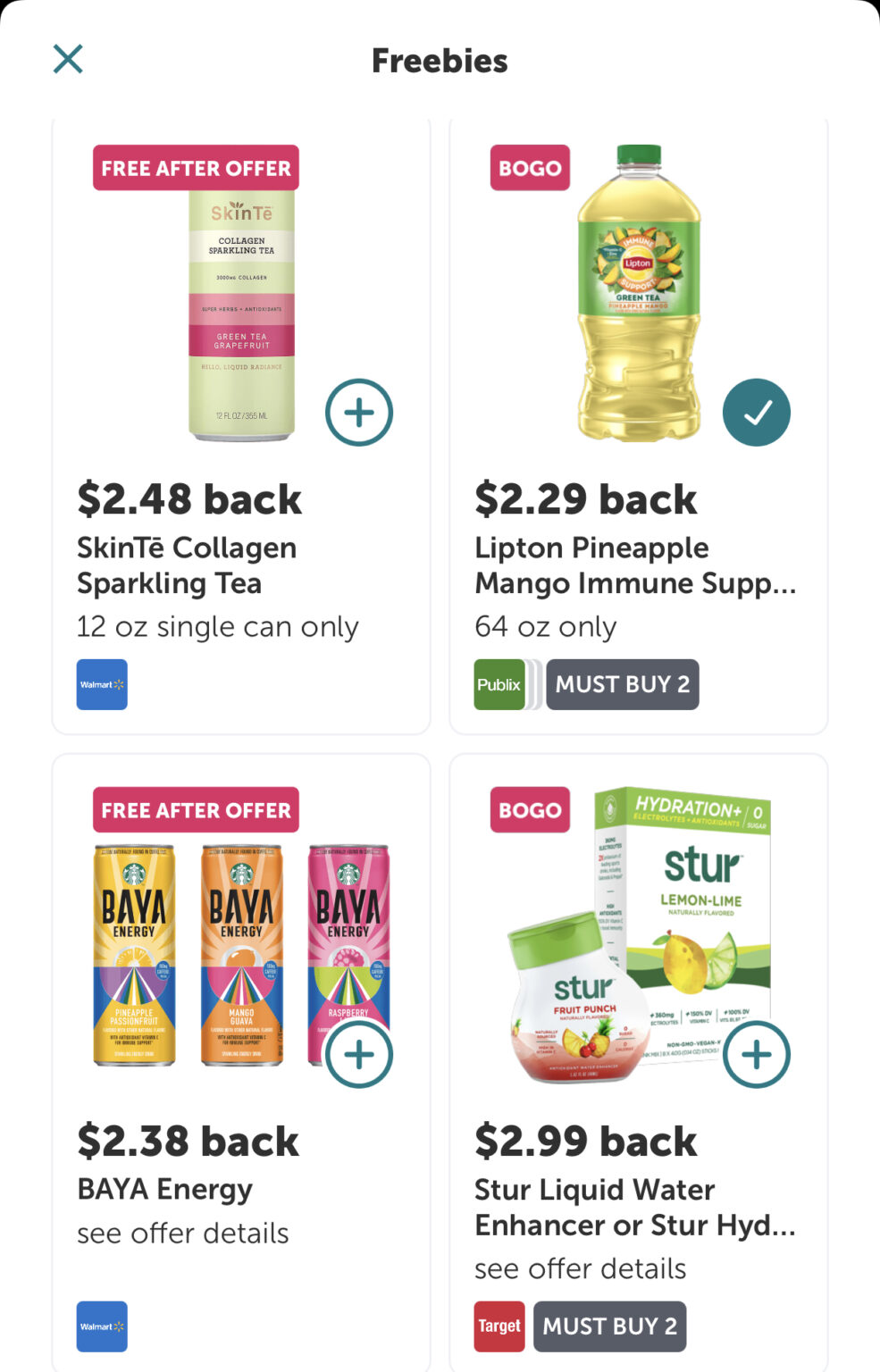This screenshot features four distinct product promotions across various stores. The first product is Skin Tea Collagen Sparkling Tea, with a cashback offer of $2.48. The second product is Lipton Pineapple Mango Immune Supporting Tea, which offers $2.29 cashback per unit and requires the purchase of two to be eligible for the deal, effectively making it free after the offer. The third product is Baya Energy Drink, with a cashback offer of $2.38. Lastly, there is a BOGO (Buy One Get One Free) deal for Stir Liquid Water Enhancer, available in Lemon Lime and Fruit Punch flavors, with a cashback offer of $2.99, also requiring the purchase of two.

Each of the four products is marked with a turquoise circle containing a symbol: Skin Tea Collagen Sparkling Tea, Baya Energy Drink, and Stir Liquid Water Enhancer all feature a turquoise plus sign, while Lipton Pineapple Mango Immune Supporting Tea features a turquoise circle with a white check mark. The cashback offers are available at different stores: Target, Publix, and Walmart, respectively.